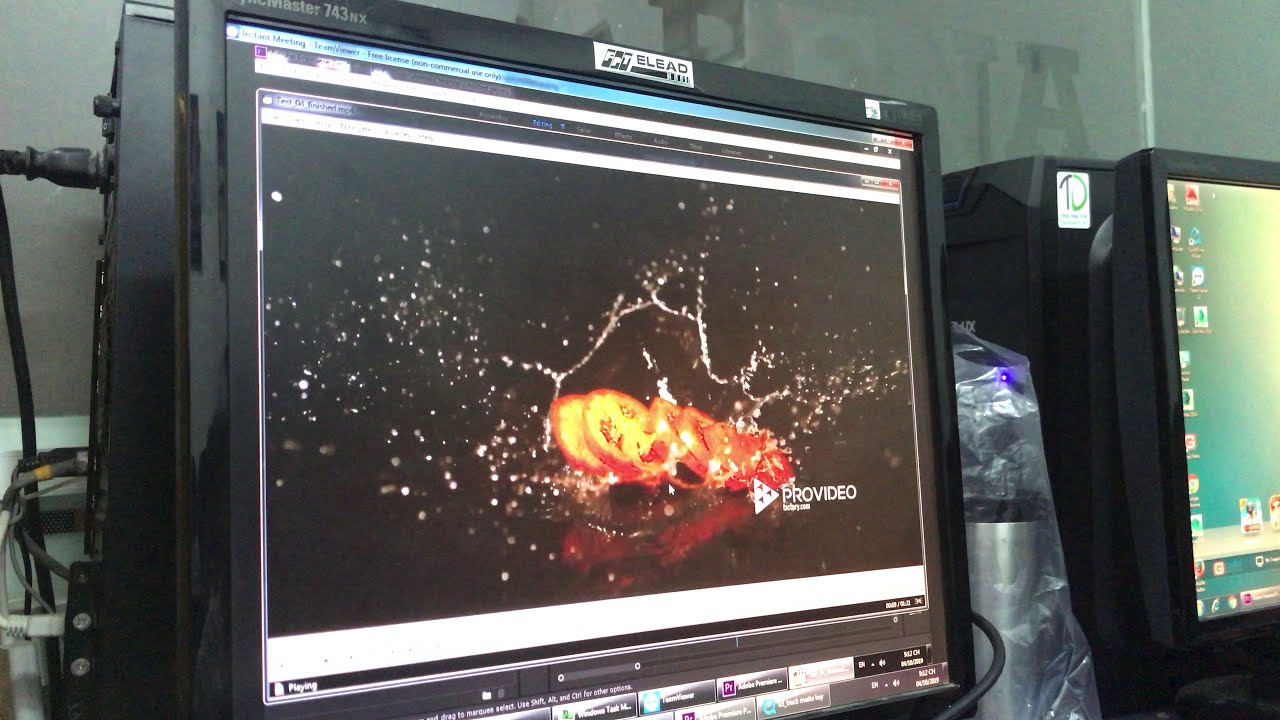The image displays a prominent computer screen showcasing a vivid image of sliced tomatoes on a black surface with water splashing around them. The bottom right corner of this screen features the label "pro video" accompanied by a white triangle logo. Adjacent to this primary screen, there is a partially visible second monitor displaying a desktop with a blue and yellow gradient background and various icons. Positioned to the right of the main screen, you can see a stainless steel tumbler and a plastic bag. The setting appears to be indoors, possibly a workspace or a warehouse, with visible cables and cords around the monitors against gray walls.